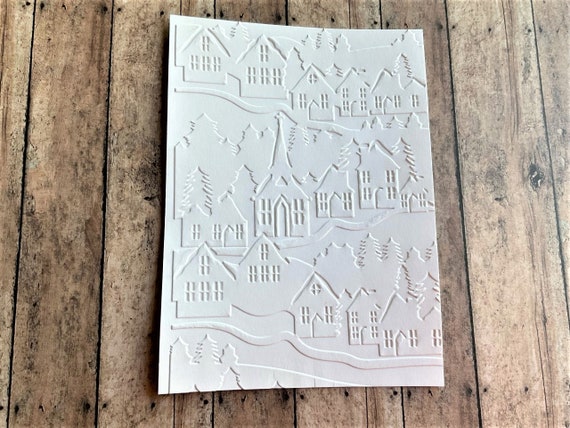The outdoor color photo showcases a white embossed piece of paper, featuring an intricate scene of a quaint, old-time village. The village, reminiscent of a charming Christmas card, displays two-story cottages, a central church, and evergreen trees. The detailed embossing captures homes, trees, and possibly rivers on a hilly landscape with pine trees in the background. The edges of the paper are somewhat warped, indicating wear, with slight curling visible. This delicate paper sits atop a rugged wooden surface, possibly a bench or table with visible nail holes and wood knots, offering a striking contrast to the pristine white embossing. The raised parts of the embossed image suggest it might be used for creating designs by rubbing a pencil or crayon over it to transfer the scene onto another surface.